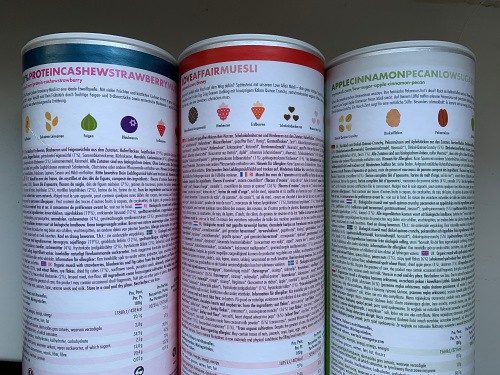The image depicts three cylindrical containers reminiscent of Pringles cans, arrayed against an off-white wall that gradually transitions to a darker gray at the top. Each canister features a unique colored border and distinct labeling. 

- The can on the left is distinguished by its blue border and is labeled "Protein Cashew Strawberry." It showcases images of strawberries, blueberries, seeds, and other ingredients. Although the can evidently contains detailed ingredient and nutritional information, the print is too small to decipher.

- The central can has a striking red border and bears the label "Love Affair Muesli." Similar to the first, the print on this can is too small to read beyond the main label.

- The can on the right, edged in white, reads "Apple Cinnamon Pecan Low Sugar." Again, the additional text is obscured due to its minuscule size.

The composition and variance in labeling suggest a collection of health-oriented, perhaps artisanal food products, each offering different flavor profiles and dietary benefits.